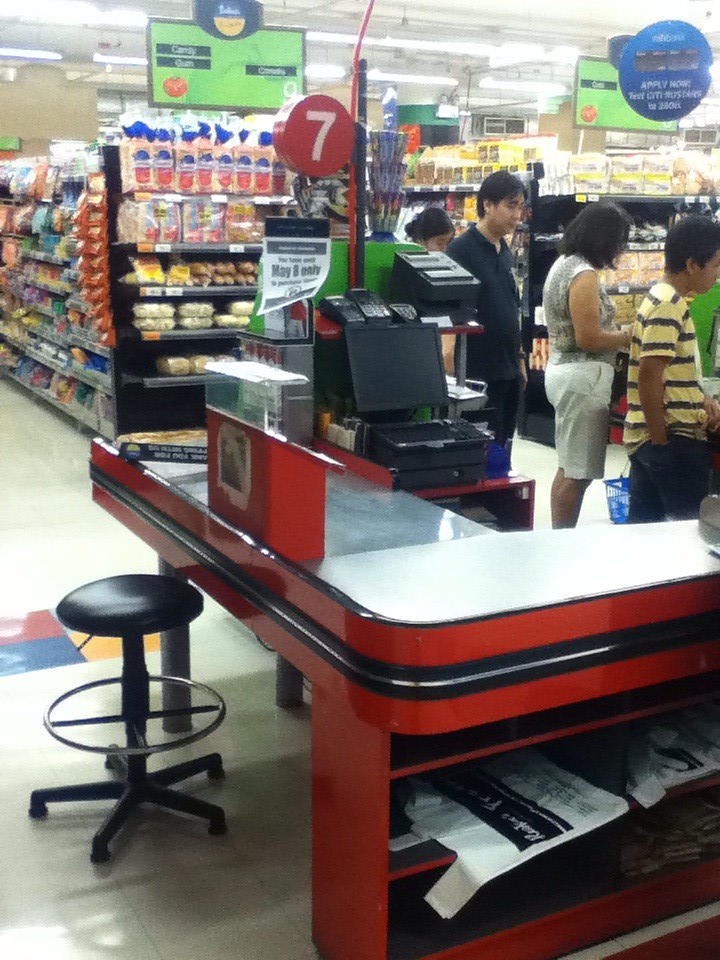The image is a highly detailed color photograph taken inside a well-lit supermarket or grocery store, likely in Asia. In the foreground, an unused checkout lane labeled with a large white number 7 atop a round sign on a pole is prominently featured. This checkout consists of a sleek silver stainless steel top with a red stand encompassing a black protective band, accented by a silver bead running horizontally through the center. A black stool with a cushioned seat and a downward-pointing gas lift lever is positioned next to the checkout.

The cash register on this lane is black and currently turned off, with credit card machines visible near the top. A flyer announcing a "May 8th party" is also notable in this area. Behind the empty checkout, packed aisles filled with various packaged food items stretch into the background, with some aisle end caps designated for refrigerated goods.

To the right of the image, several people—an Asian man in a t-shirt, a woman in shorts and a tank top, a child in a yellow and black striped shirt, and a man in a black shirt—are standing in line, queuing for another checkout that is partially visible. Large green signs above the aisles and a prominent blue sign reading "Apply Now" contribute to the vibrant color scheme, which includes red, green, and other bright hues.